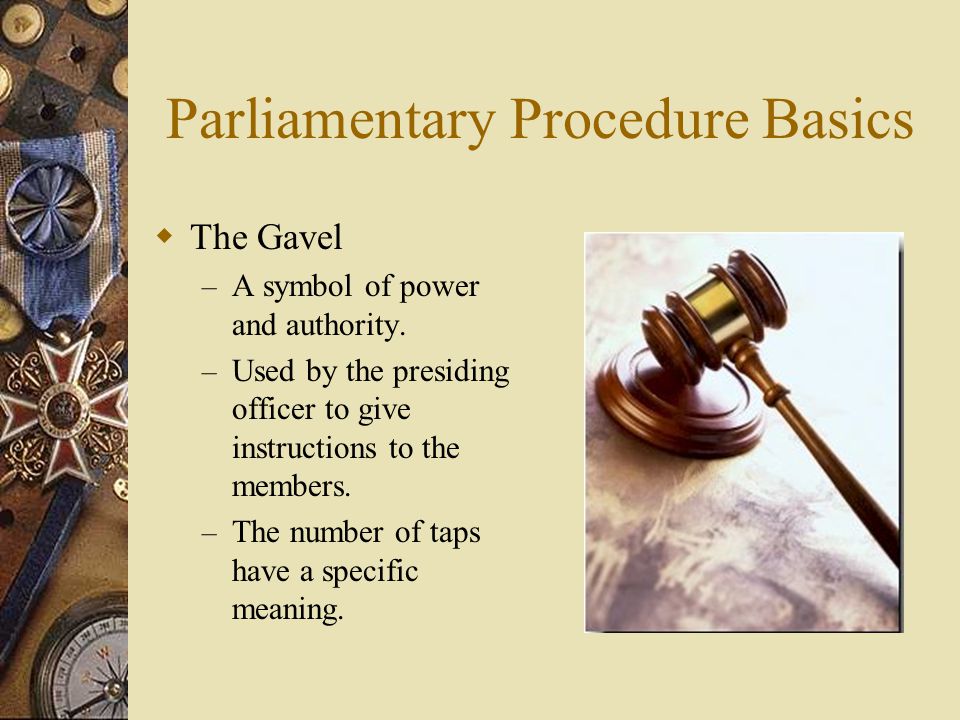The image is an informative slide presented in landscape orientation, primarily designed as an infographic. The background is a beige color, and it prominently features the title "Parliamentary Procedure Basics" in gold text at the top. On the right side of the image, there is a detailed photograph of a wooden gavel with a brass band around its handle, resting on a round wooden base placed on a white tablecloth. This gavel, a symbol of power and authority, is situated slightly to the right of the image’s center.

On the left, there is a decorative border adorned with gold medallions and an assortment of radial dial emblems. Alongside these emblems, there are several notable insignias including a compass, a badge, and a ribbon, with one emblem featuring a cross encompassed by four red triangles.

Centrally displayed are three text points highlighted under a gold diamond-shaped bullet, explaining the gavel's significance: "A symbol of power and authority," "Used by the presiding officer to give instructions to the members," and "The number of taps have a specific meaning." This slide combines elements of realism through its detailed photography and a structured graphic design, making it visually engaging and informative.